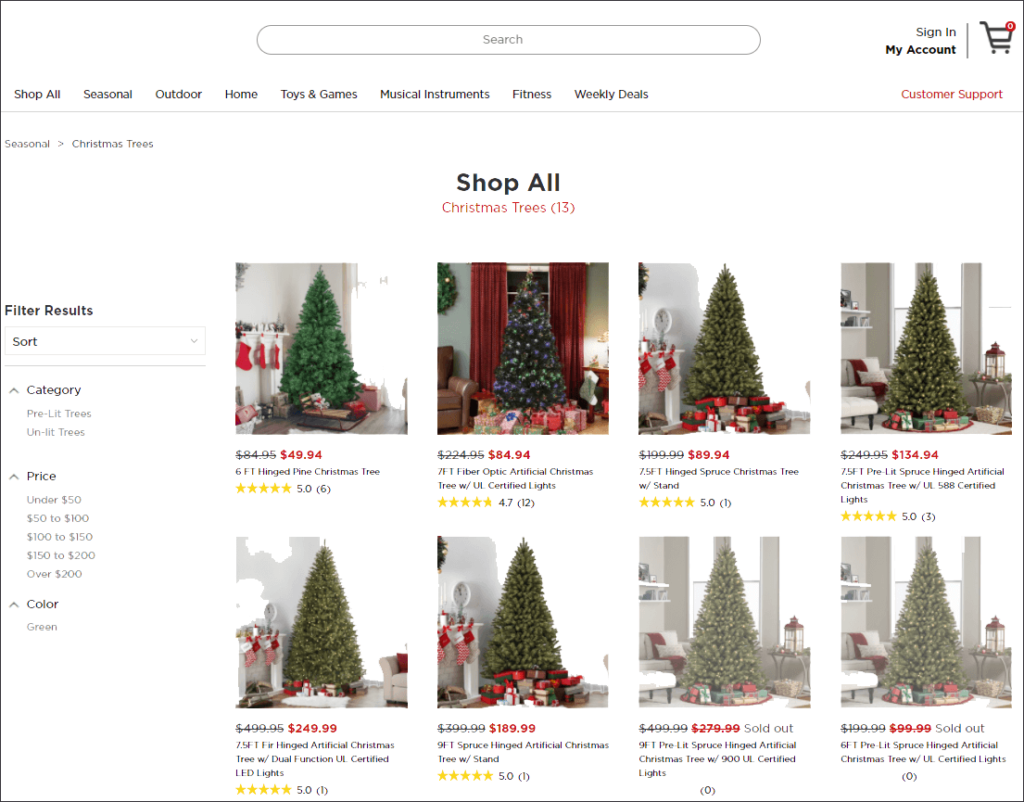The webpage features an online store that sells various goods and products. At the very top, there is a long, oval-shaped search bar centered with the word "Search" within it. To the right of the search bar, there are options for "Sign In" and "My Account", followed by a thin line divider and a shopping cart icon with a small circle on top.

On the left-hand side of the page, there is a vertical menu featuring categories such as "Shop All," "Season," "Outdoor," "Home," "Toys and Games," "Musical Instruments," "Fitness," and "Weekly Deals." 

On the right-hand side, in red font, is a "Customer Support" link, separated by another thin line. Below this, in bold, the text reads "Shop All," followed by a subcategory in red font for "Christmas Trees" with a number "13" next to it, indicating the number of products available. 

The page showcases eight artificial Christmas trees, each accompanied by ratings and prices listed as follows:
- $49.94
- $84.94
- $89.94
- $134.94

Below these items, the prices continue for additional products outside the visible range in the image. On the left-hand side, there is a "Filter Results" section, which includes options to sort by a drop-down arrow, categories with various items, a price range, and one color option listed as "Green."